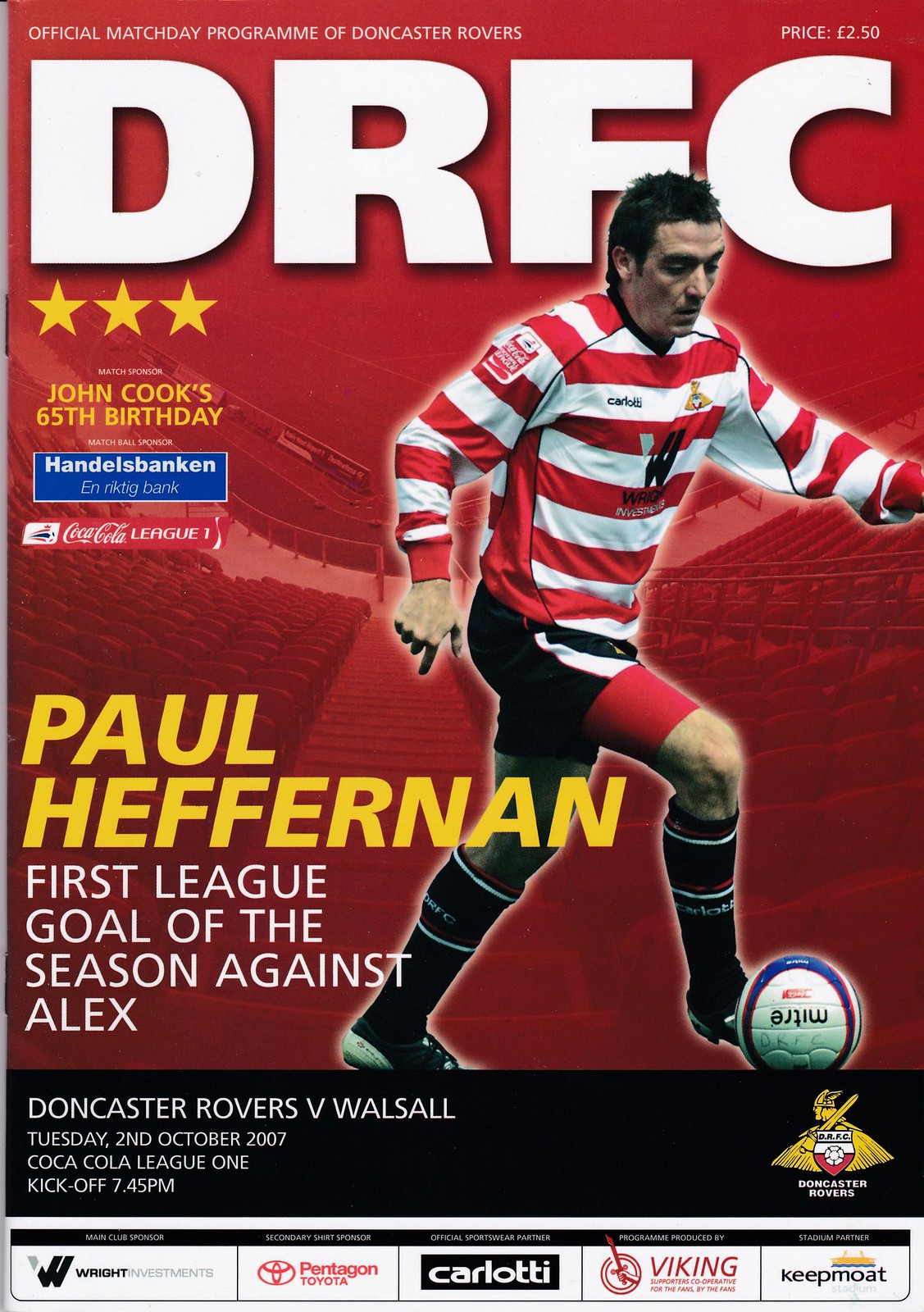The cover of the DRFC official matchday program for Doncaster Rovers, priced at £2.50, vividly features Paul Heffernan in action. He is caught mid-motion, wearing a red and white horizontally striped jersey, black shorts with red undershorts, black knee-high socks, and black shoes. At his foot is a white soccer ball emblazoned with "MITRE" and decorated with red and blue circular lines. In large white letters at the top, it says "DRFC," with the small print above stating it's the official match day program. The background is predominantly red, depicting the stadium's bleachers.

To the left of the player are three yellow stars, alongside a yellow tribute to John Cook's 65th birthday and the name Paul Heffernan in golden print. Below it, in white, it reads "First league goal of the season, against Alex." Notable sponsors such as Coca-Cola League and Handelsbanken feature prominently. 

The bottom of the cover details the match specifics: Doncaster Rovers vs. Walsall, Tuesday, 2nd October 2007, Coca-Cola League 1, kickoff at 7.45 p.m. The Doncaster Rovers logo, with a gold Viking wielding a sword in front of a red and white shield, is positioned on a black footer alongside various sponsor details.